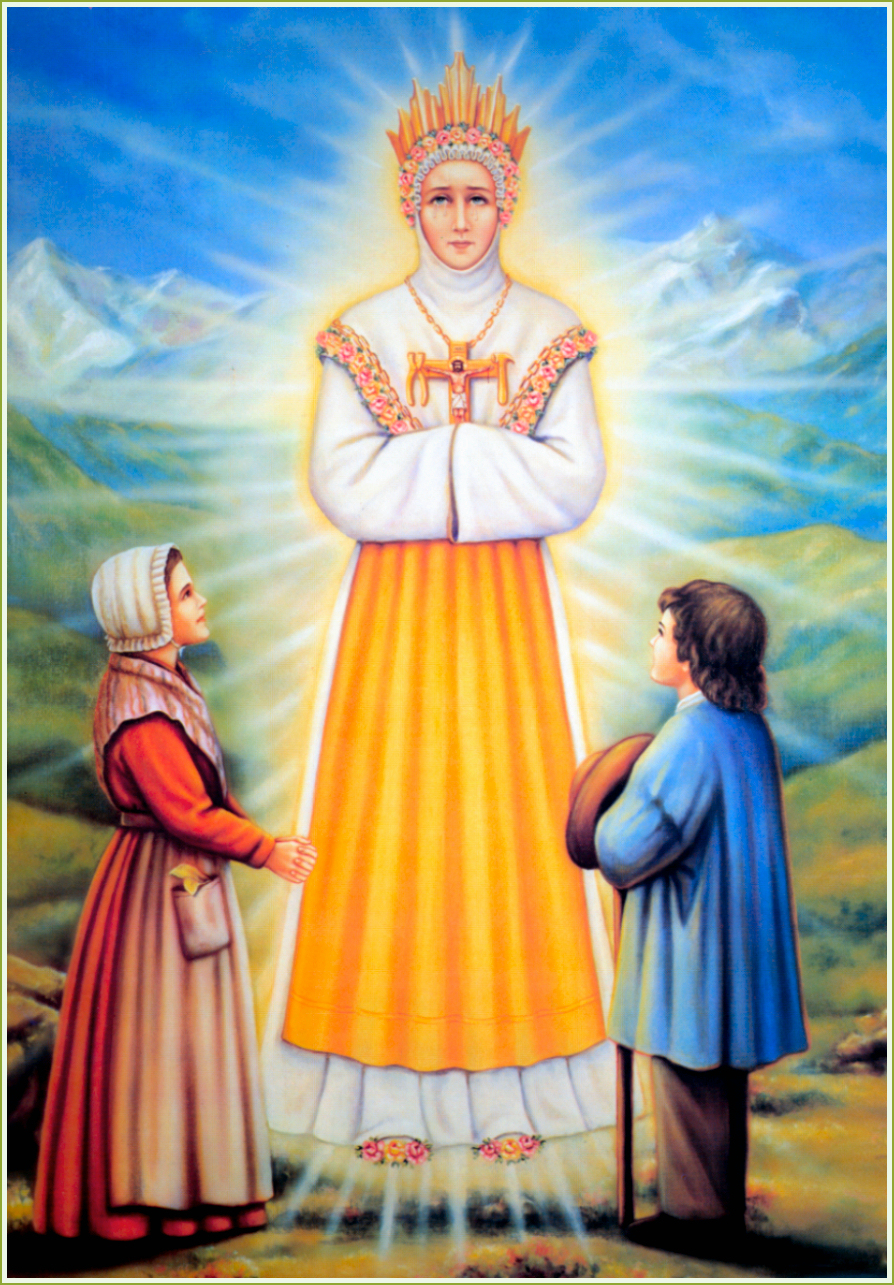The painting depicts a holy woman, perhaps an angel or saint, centered within the composition. She is adorned in a white robe with an orangish-yellow apron and a prominent golden cross necklace. A glowing aura of white and yellow light radiates from her, enhancing her divinity. She wears a golden crown and keeps her hands modestly hidden within her sleeves. Flanking her are two children rendered in vivid attire: a girl on the left in a red and white dress with a head covering, and a boy on the right holding a hat and possibly a walking stick, garbed in blue. Both children gaze up at the central figure with expressions of awe and excitement. The background showcases a serene natural landscape with green hills, a valley, white-peaked mountains, and a bright blue sky, suggesting a medieval or Renaissance setting.